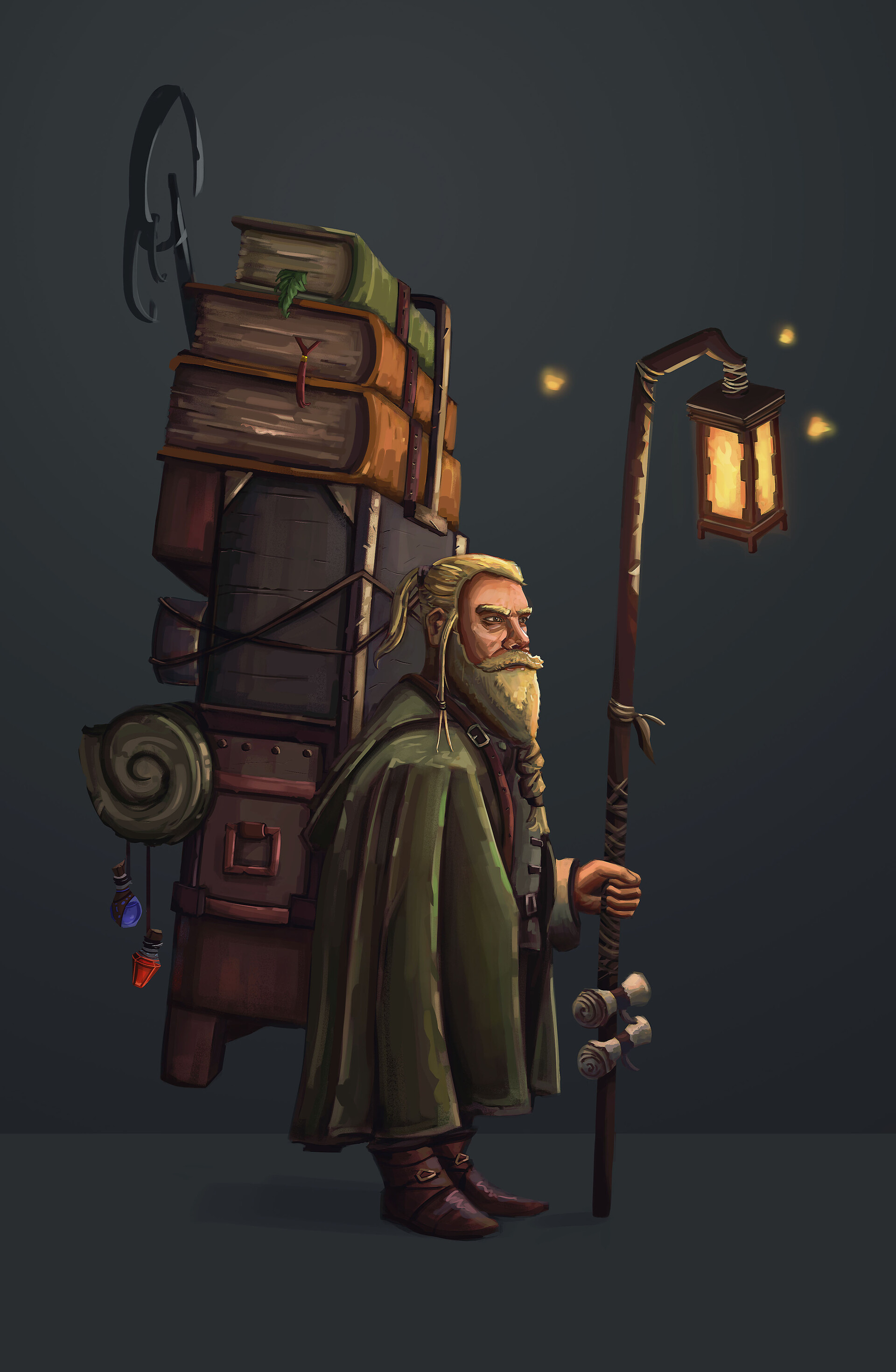The image is a whimsical, detailed cartoon illustration of an older man with a medieval, Viking-like appearance. He stands in a dark, nighttime setting, illuminated only by a lantern he holds on a pole in his left hand. The man's long, blonde hair is tied into a neat ponytail, and his massive beard, which extends to his chest, is also meticulously tied and rolled. He sports very thick eyebrows and brown boots, and he is draped in a dark green cape that adds to his old-world charm.

This quirky character is burdened with an exaggeratedly large backpack that towers over his head, filled with an assortment of items. The backpack is an impossible mix of a massive trunk, a rolled-up blanket, a piece of furniture, and three enormous books. Sticking out from the backpack is also some sort of wheel or netting, adding to the far-fetched nature of the illustration.

Facing towards the right of the image with a distant, serious expression, he stares into space, giving a sense of a journey or quest. Adding a whimsical touch, the lantern he holds seems to have doorknobs attached, and there are three small glowing bugs buzzing around it, accentuating the magical, fantastical atmosphere of the drawing.